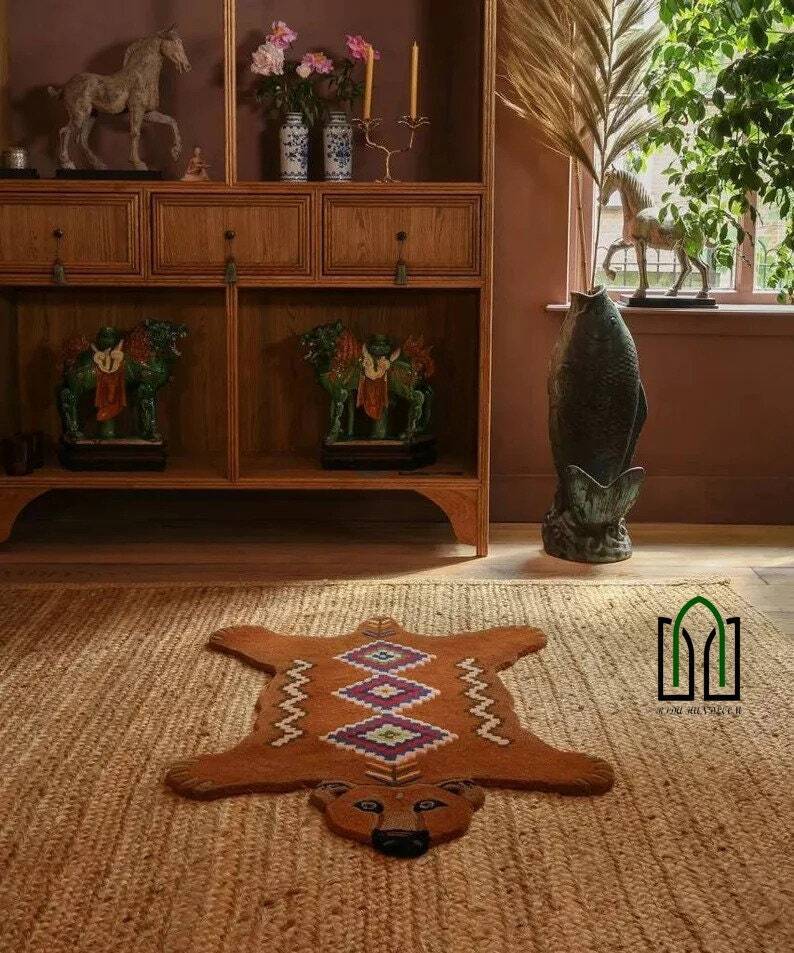The photo depicts the interior of a house featuring a rough-textured, light beige woven grass rug covering the floor. On top of this rug lies a brown animal rug, resembling a bear but clearly an imitation, which is adorned with indigenous-inspired patterns, including diamonds and zigzag shapes along its back and sides. To the left, a bookshelf with various drawers showcases an array of knick-knacks, such as a wooden horse statue and a two-candle candelabra. The bottom shelf holds additional statues. To the right of the bookshelf stands a fish-shaped vase with a vibrant green plant emerging from its mouth. In the bottom right corner of the image, a logo is visible.